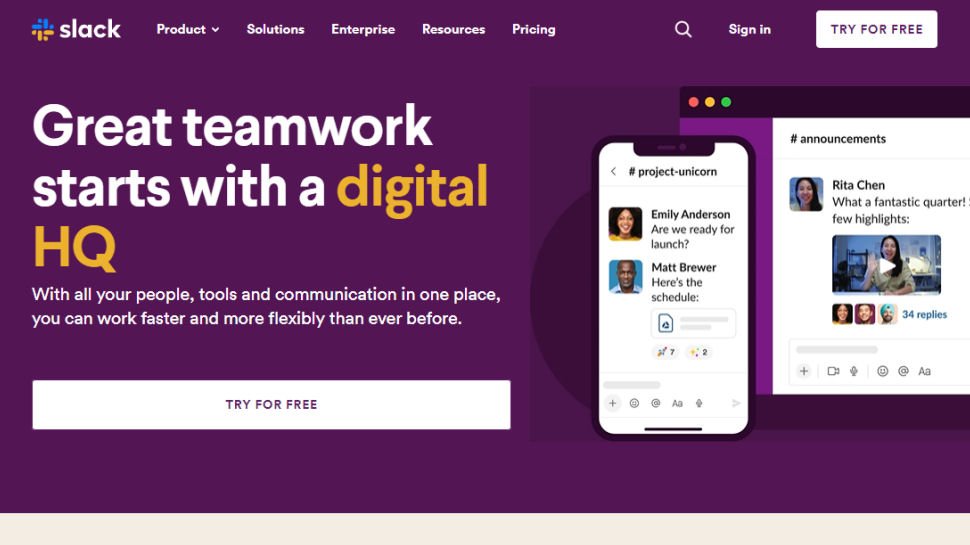The upper left corner of the image features the Slack logo, characterized by its intricate design: a cross-like structure where the top half is blue and the bottom half forms a plus sign with blue and orange hues interwoven. Adjacent to the logo, the navigation bar displays options such as "Product" with a drop-down menu, "Solutions," "Enterprise," "Resources," "Pricing," a magnifying glass icon, "Sign In," and a "Try for Free" button. The background of this header section is a deep purple shade, while most of the text is rendered in white.

Prominently displayed on the left side of the image is a bold headline reading, "Great teamwork starts with a digital HQ," with "Digital HQ" highlighted in orange and blue, in large font. Below the headline, smaller text elaborates: "With all your people, tools, and communication in one place, you can work faster and more flexibly than ever before." Beneath this text is a prominent white button with "Try for Free" written in purple.

On the right side of the image, a tablet and a cell phone display interactive Slack messages. The cell phone screen shows a conversation under the hashtag #projectunicorn with Emily Anderson asking, "Are we ready for launch?" and Matt Brewer replying, "Here's the schedule." The tablet screen features a channel called #announcements, where Rita Chen exclaims, "What a fantastic quarter," followed by "Few highlights" and a note of 34 replies. The overall color palette of the image incorporates purple, yellow, blue, white, and orange tones.